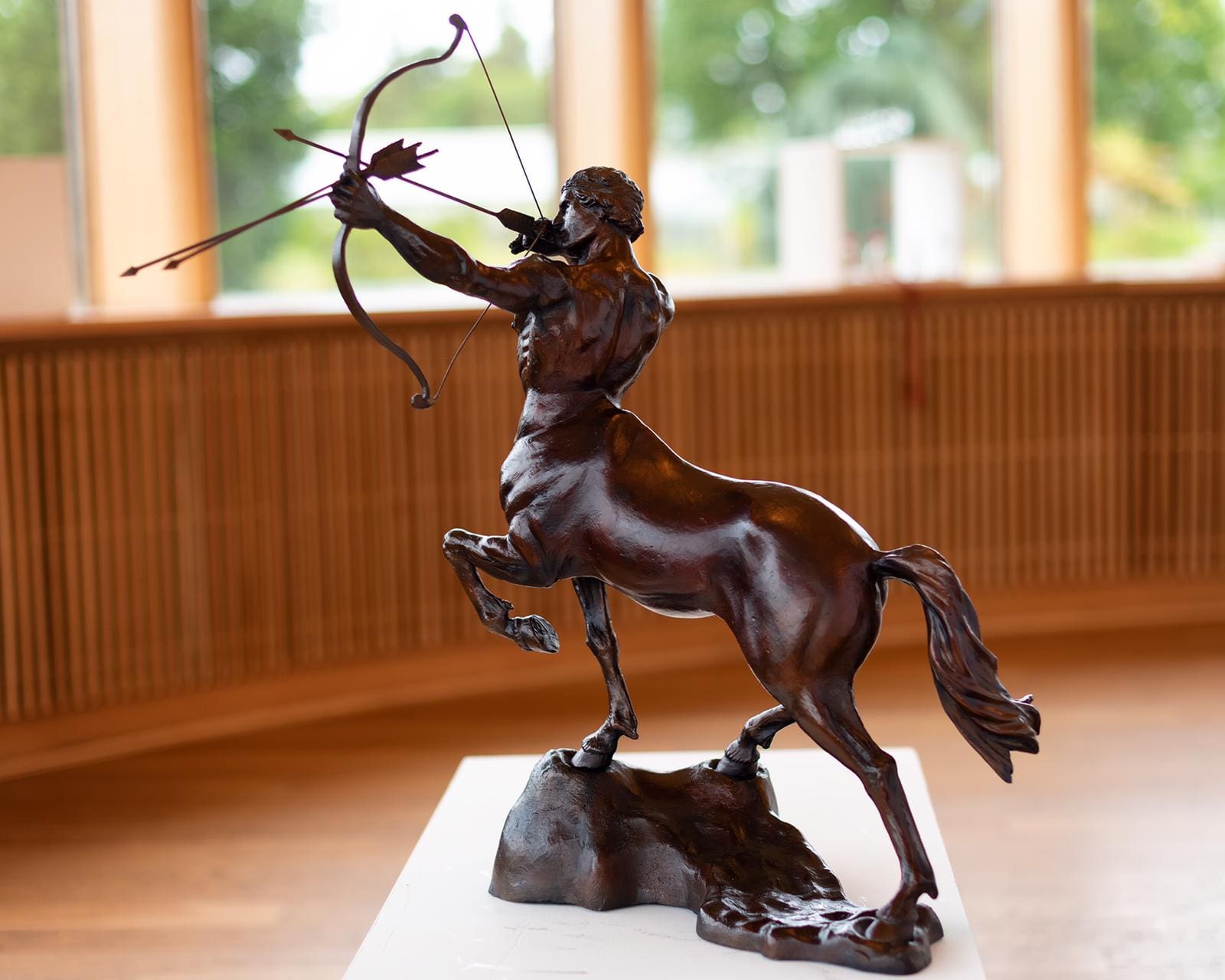This image showcases a detailed close-up of the Archer Centaur sculpture by Irish sculptor Michael Keane. The sculpture, centered sharply in the frame, is brown in color and depicts a centaur—a mythical creature that is half man, half horse. The top part of the sculpture is a muscular man pulling back an arrow in his bow, poised to shoot. The lower part transitions into the body of a horse, complete with a tail and depicted as if standing on a rocky base, which rests on a white mat. The background, which is out of focus, features a wooden floor and railing, along with windows revealing a green area outside. Additionally, there are orangish pillars flanking the sculpture, contributing to a setting that resembles a museum or gallery.